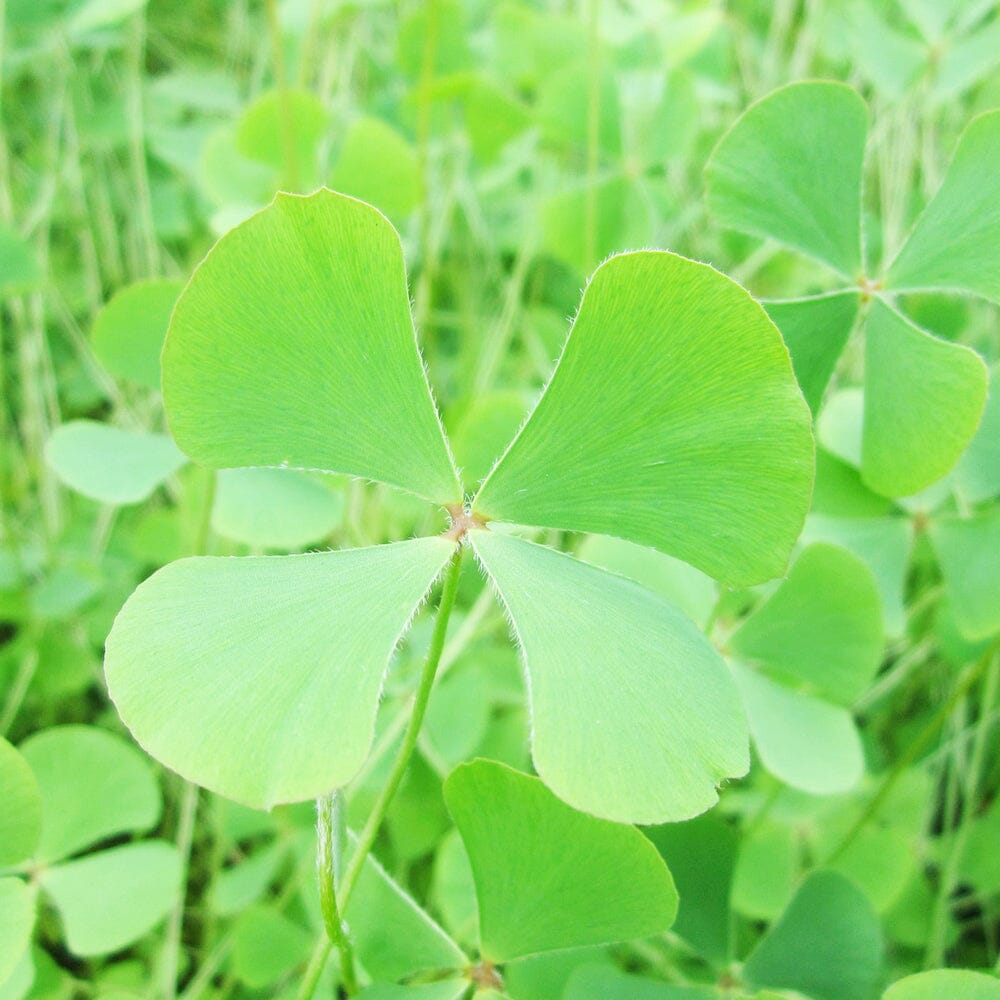This detailed close-up photograph showcases a vibrant field of four-leaf clovers in a striking leprechaun lime green. In the foreground, a prominent four-leaf clover reveals leaves that are about four to five inches long and slender, accompanied by a long stem. The fine hairs on the leaves highlight the sharpness of the clover in focus. Scattered throughout the image, multiple four-leaf clovers can be observed, although some are out of focus and located towards the upper right and bottom right corners of the frame. The blurred background suggests an expansive field filled with more of these rare clovers, characterized by their similar size, color, and clustered green stems that add a delicate texture to the composition. This panorama creates an impression that the field is entirely comprised of four-leaf clovers, although the details grow softer as the eye moves towards the horizon.